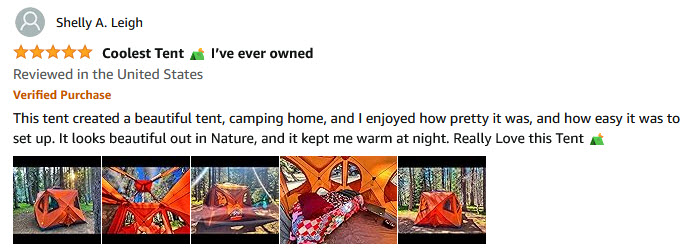**Detailed Caption:**

This image appears to be a screenshot from a website, likely an Amazon review. The background is white with predominantly black text. In the upper left corner, there is a grey person icon resembling a circle with a head and shoulders in a lighter grey shade. Beside the icon, the name "Shelley A. Lee" is displayed, accompanied by five orange stars indicating a five-star rating. 

Underneath the name and stars, there is a headline that says, "Coolest tent," followed by a small tent icon or emoji. This review is for a tent, noted as being reviewed in the United States and marked as a verified purchase. The main body of the text reads: "This tent created a beautiful tent camping home, and I enjoyed how pretty it was and how easy it was to set up. It's beautiful out in nature and kept me warm all night. Really love this tent," followed by another tent emoji.

The review includes a series of five images showcasing the tent. The first, third, and last images display black bands at the top and bottom, each illustrating different views of the tent. The first image shows the tent pitched among trees on the left-hand side. The second image offers a close-up view, depicting the tent with cartoon-like features including eyes, a nose, and ears. The third image portrays the tent from a distance, set against a wooded background. The fourth image provides an interior view of the tent, featuring orangish walls and some bedding. The fifth image captures the tent again in a woodland setting with sunlight illuminating the grass in the background.

Overall, the photos are quite small, making it challenging to discern finer details.